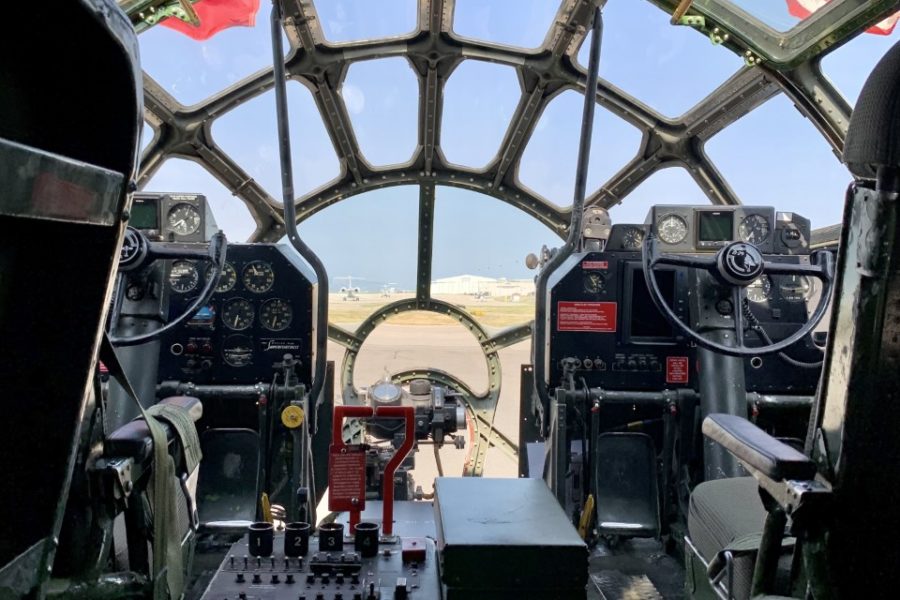This high-quality photograph captures the interior of the iconic Millennium Falcon cockpit from the Star Wars franchise. The image is taken from a perspective behind the two pilot seats, looking out through the glass-domed front windows. The cockpit's unique design features metal frames and segmented glass panes that wrap around the front, reminiscent of the starship’s famous look. Each pilot seat is equipped with a semi-circular steering wheel and an intricate gauge panel. Between the seats lies a set of handles that control the starship. A red lever is distinctly positioned to the right of the left seat. The cockpit floor reveals foot pedals used to maneuver the vessel. In the distance, through the glass panels, other Star Wars ships can be seen parked in a desert-like setting, with a backdrop of golden dirt, scattered brush, a white building, and a light blue sky. The detailed and immersive setup evokes the grandeur and adventure of the Millennium Falcon as it prepares for its next journey through space.